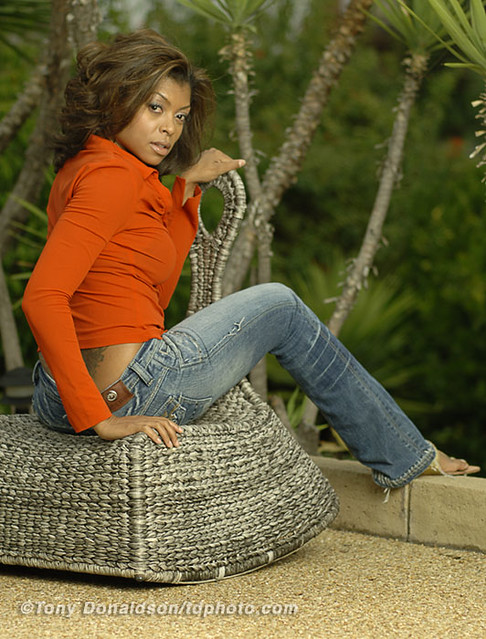The image portrays a multicultural woman with dark hair, sitting on a unique stool-like chair made of grey jute, rather than a traditional chair. She is wearing jeans and either barefoot or donning very skimpy sandals. Her red shirt, tied around the waist and accompanied by a belt, exposes a tattoo on her back. The woman sits on the chair leaning slightly to the right while her face is turned toward the camera, giving her an engaged look. The paved path beneath her is light brown and appears sandy. The background is lush and filled with greenery, though it is blurred to emphasize the woman in the foreground. Text at the bottom of the image reads “tony donaldson / tdphoto.com.”